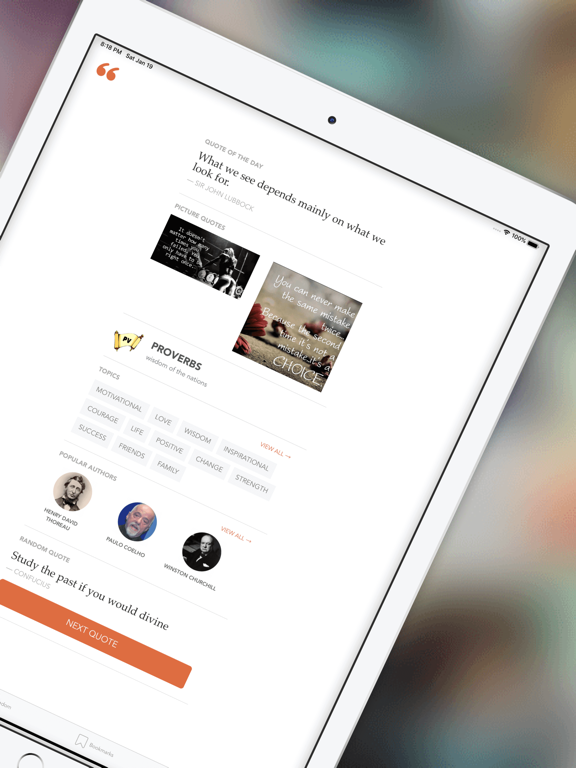This image displays a white Apple iPad angled slightly, showing its screen which features a white webpage. At the top left of the iPad's screen, there's a pair of quotation marks icon, highlighting the section titled "Quote of the Day." Centrally, the quote reads: "What we see depends mainly on what we look for." The author of the quote is listed directly below this text.

Further down the screen, there are two small thumbnail images labeled as "Picture Quotes," with one picture quote positioned on the left and another on the right. Underneath these thumbnails, the heading "Proverbs" appears, followed by the partially blurred text that reads "Wisdom of the..." due to its small size.

Proceeding further, there is a section dominated by a series of gray boxes containing various tags. The heading "Topics" is placed above these tags, and to the right, the option "View All" is highlighted in red. Below this section, the heading "Popular Authors" is displayed, featuring circular profile pictures of different authors with their names printed underneath each photo. To the right of this section, another "View All" link is also visible in red.

Near the bottom of the screen, there's a segment titled "Random Quote" displaying the quote: "Study the past, if you would divine the future," with the author's name attributed at the bottom. Lastly, at the very bottom in a prominent orange color, there is an option labeled "Next Quote."